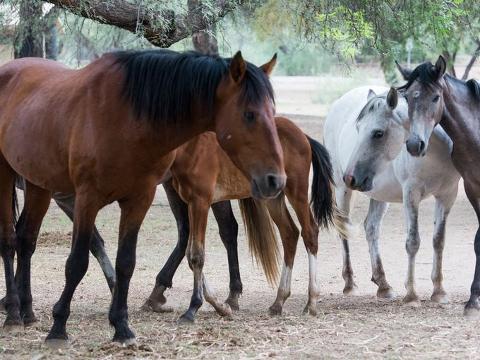In this detailed outdoor photograph, a small group of horses and foals are gathered, totaling at least five, some partially obscured. Dominating the image is a large chestnut-colored horse on the left, identifiable by its flowy black mane and dark eyes, with its head turned slightly right and a hint of white around its nostrils. Nestled beside it, a smaller lighter chestnut foal is nearly hidden, showing only four slender legs and a black tail. Behind these, the legs of another horse are visible, but its details remain unclear. To the right, a more defined smaller white horse with a gray nose and ears stands out, head turned left towards the prominent chestnut horse. Lastly, a grayish dappled horse, exhibiting a bit of white on its forehead and a mane cascading over its face, completes the scene on the far right, partially moving out of the frame. The setting is enhanced by hay-littered ground and majestic large trees draped in Spanish moss, casting a serene, pastoral backdrop.